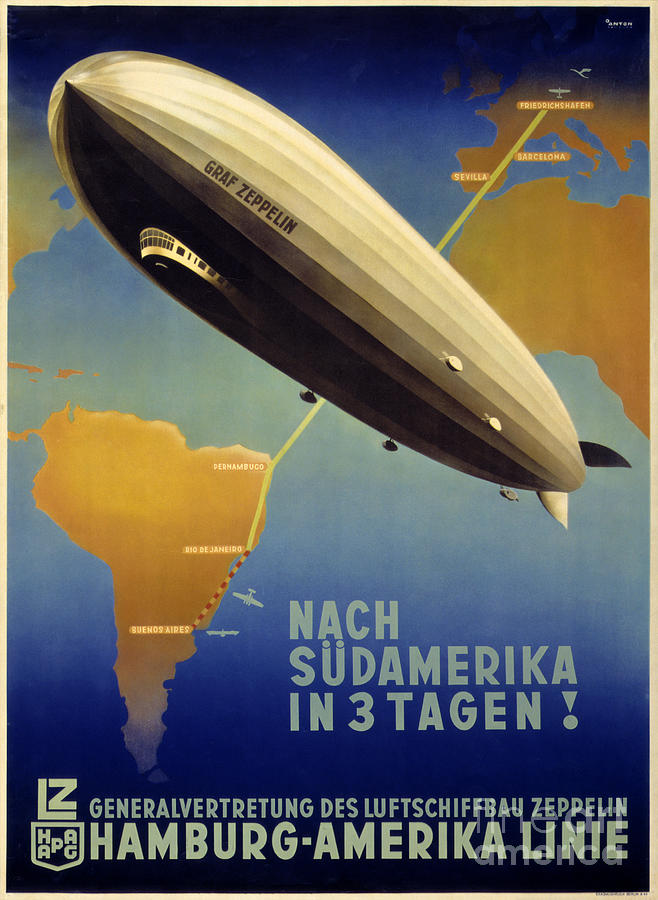The image depicts a vintage propaganda poster featuring a large tan-colored zeppelin with a darker brown underbelly labeled "Graf Zeppelin." The zeppelin is centered and facing towards the top left corner. Below the airship, there's text in German, "Südamerika in drei Tagen!" with an exclamation mark. Behind the zeppelin, a stylized map is visible, designed in a watercolor painting style, which shows parts of South America, North America, Europe, and Africa. Cities in both Europe and South America are marked, and these cities are connected by a yellow line, resembling a flight path. Additional German text blocks are scattered around the map, with a notable section of text near South America and another label towards the left. An observation area is visible underneath the zeppelin, suggesting a place for passengers. The overall aesthetic of the image is classical, likely intended to evoke a nostalgic or historical sentiment.